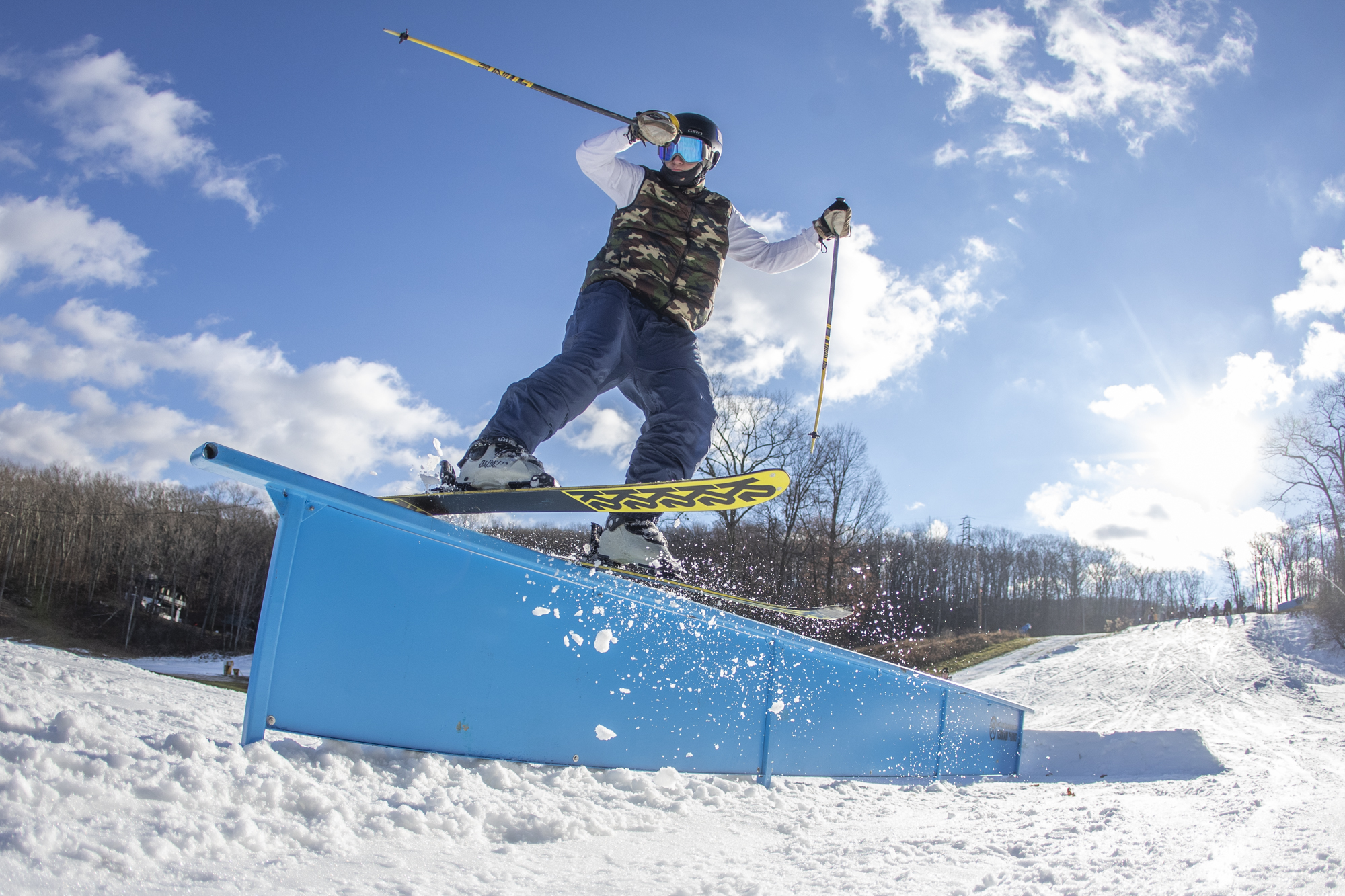In this vibrant photograph, a skier is captured mid-jump over a blue barrier that stretches horizontally across the snowy downhill slope. The skier, equipped with a yellow snowboard, dons snow goggles, a ski mask, and a helmet. He wears a green and white print ski jersey over a white shirt, blue ski pants, and white boots attached to the skis. The scene is set on a bright day, with a pale sun shining from the right, illuminating a light blue sky dotted with puffy white clouds. Bare trees, devoid of leaves, frame the snowy hill on both sides, enhancing the wintry ambiance. Snow flurries off the skier's skis, highlighting the dynamic motion as he soars over the barrier.